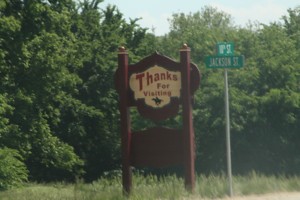The photograph captures the rear view of a wooden sign set at the corner of an intersection, marking the exit of a park or city. The primary message on the sign reads "Thanks for visiting," suggesting that travelers are departing from the location. It's logical to infer that the front side of this sign might greet newcomers with a "Welcome to [Location]" message. The sign is anchored by two sturdy wooden posts and features an intricately carved upper section where the farewell message is displayed. Below this main sign, there is a secondary, smaller sign that is blank from this perspective.

The setting of the sign is in a grassy area adjacent to the road, surrounded by a dense, wooded area that extends into the background. The intersection itself is denoted by a street sign that reads "Jackson Street" and another sign which possibly indicates "10th Street." The sky is partially visible through the treetops, contributing to the serene atmosphere of the scene. The combination of the rustic wooden sign and the lush, natural surroundings creates an inviting yet nostalgic visual experience for those passing by.